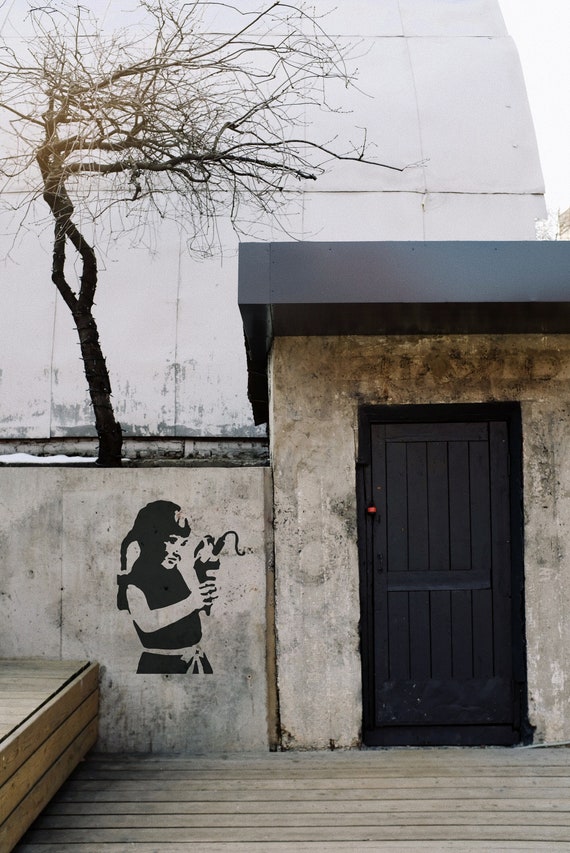The image captures the entrance of a concrete building, styled to resemble street art and urban decay. The entryway, featuring a wooden floor made of slats, leads up to a black-painted wooden door framed by concrete and topped with a black metal overhang. To the right of the doorway, a wooden bench complements the scene. Adjacent to this, on the left, is a large wall bearing a provocative decal: an edgy black stencil of a joyful little girl with pigtails. She's holding an ice cream cone with a stick of dynamite in it, an ironic and dangerous twist that mimics the style of Banksy. Above the stencil, there's a sparse, leafless tree, emphasizing the decay and contrasting with the vibrant life suggested by the girl. The detailed use of negative space in the stencil incorporates the building's natural shadows and highlights, creating depth. Overall, the image blends elements of street art and urban landscape, making a bold statement.